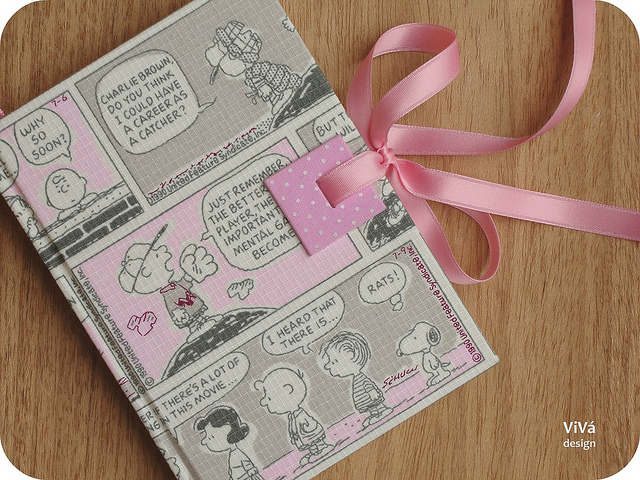This colored photograph depicts a hardcover children's book featuring a Charlie Brown comic strip on the cover. The comic, rendered in shades of gray, white, and pink, shows five panels with Peanuts characters. In the upper left, Charlie Brown and Linus are at the wall, with Charlie asking, "Why so soon?" Adjacent, on a baseball diamond, a catcher asks, "Charlie Brown, do you think I could have a career as a catcher?" The central panel shows Charlie Brown on the pitcher’s mound, saying, "Just remember, the better player the important mental game becomes," though part of the text is obscured by a small pink gift tag with white polka dots, which is attached to a pink ribbon tied around the book. At the bottom, there are four characters, including Snoopy, with Lucy speaking, "There's a lot going on in this movie," followed by Snoopy's remark, "Rats." This book, possibly resembling a diary, is placed on a light brown butcher block table, and the publisher’s mark, "Viva Design," is visible in the lower right corner.